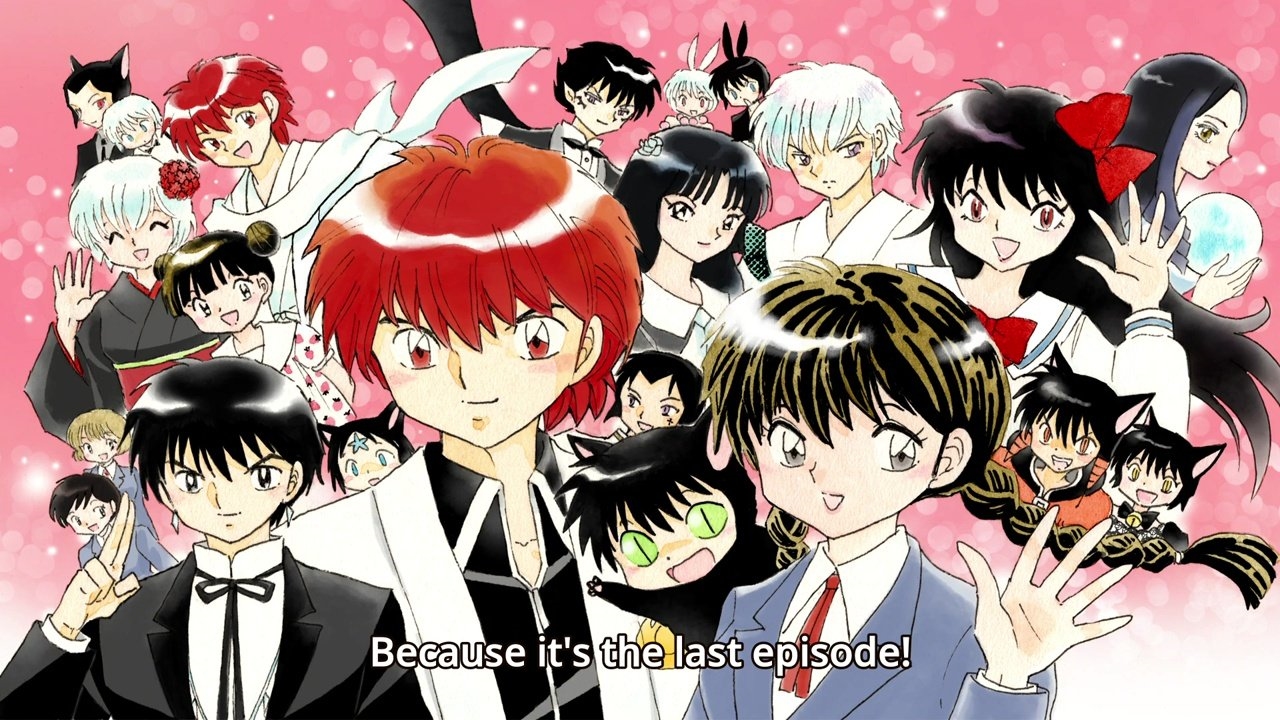This vibrant image is a celebratory scene from the Japanese anime series RIN-NE, marking the final episode. It features a diverse group of 15 to 20 anime characters, including young girls and boys, some elders, and a mix of humans and anthropomorphic beings. Two prominent figures stand in the foreground on the left: a cheerful young man with striking red hair and eyes, dressed in a black shirt with a white jacket, and a braided-haired young woman in a blue blazer, white collared shirt, and short red necktie, who raises her left hand in greeting. Surrounding them are characters sporting various attires, from school uniforms to suits and kimonos, with hair colors ranging from red and black to brown, white, and gray. Some characters sport cat ears, adding to the whimsy. The background is a pink, sparkly hue, enhancing the festive atmosphere. At the bottom of the image, the text reads, "Because it's the last episode!" in an exuberant tone.